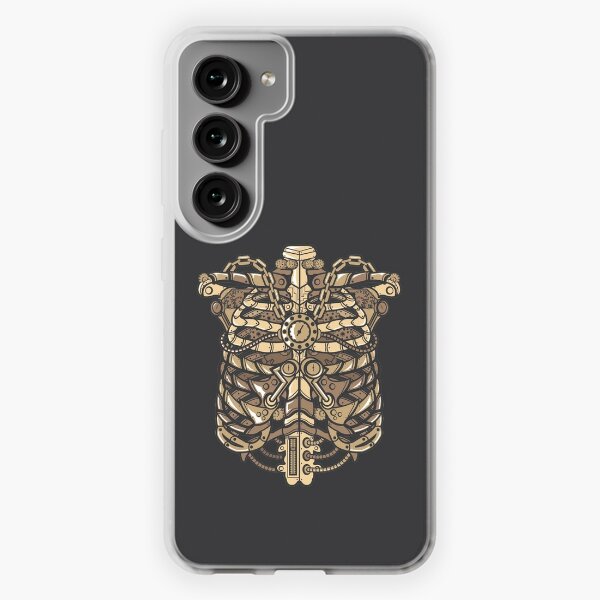The image depicts the back view of a smartphone, likely an iPhone, with a gray casing. Prominently located on the upper left corner, there are three circular black camera lenses arranged vertically, with a smaller metallic circle, possibly a sensor, to the right of the top lens. The phone rests on a white surface, emphasizing the details of its design. The back cover features an intricate graphic of a skeletal ribcage with brown hues, entwined with chains and adorned with clock-like elements and gauges. The chains wrap around the ribcage and converge in the middle of the chest area, giving the illusion of an owl face due to their arrangement. The graphic extends to the bottom, where additional circular shapes and cords are visible, contributing to the detailed and somewhat enigmatic design.